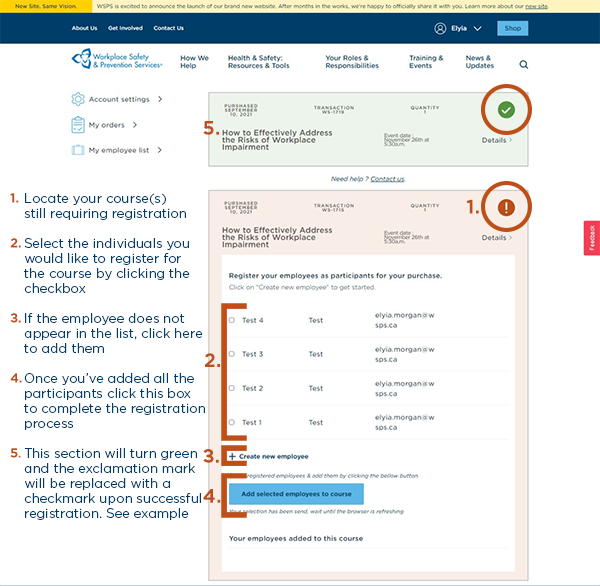The image depicts a detailed page of a Workplace website focused on safety and prevention services. At the top, there is a blue banner featuring navigation links labeled "About Us," "Get Involved," and "Contact Us." To the right, there's a user icon with the initials "DYLA," a drop-down menu, and a blue button labeled "Shop." 

Below this banner, the website's main heading, "Workplace Safety and Prevention Services," is prominently displayed against a white background. Tabs are arranged beneath this heading, including "How We Help," "Health and Safety Resources and Tools," "For Your Roles and Responsibilities," "Training and Events," and "News and Updates," accompanied by a search icon.

Directly under the main header, there are options for "Account Settings," "My Orders," and "My Employee List." 

On the left-hand side of the page, a numbered instructional section guides users through course registration:

1. Locate the course that still requires registration.
2. Select individuals to register by clicking the corresponding checkboxes.
3. If an employee isn’t listed, there’s an option to add them.
4. Once all participants are added, a box must be checked to complete the registration process.
5. Upon successful registration, the section will turn green and the exclamation mark will be replaced with a check mark, with an example provided for reference.

This website primarily facilitates the registration process for business-related safety and risk management courses.